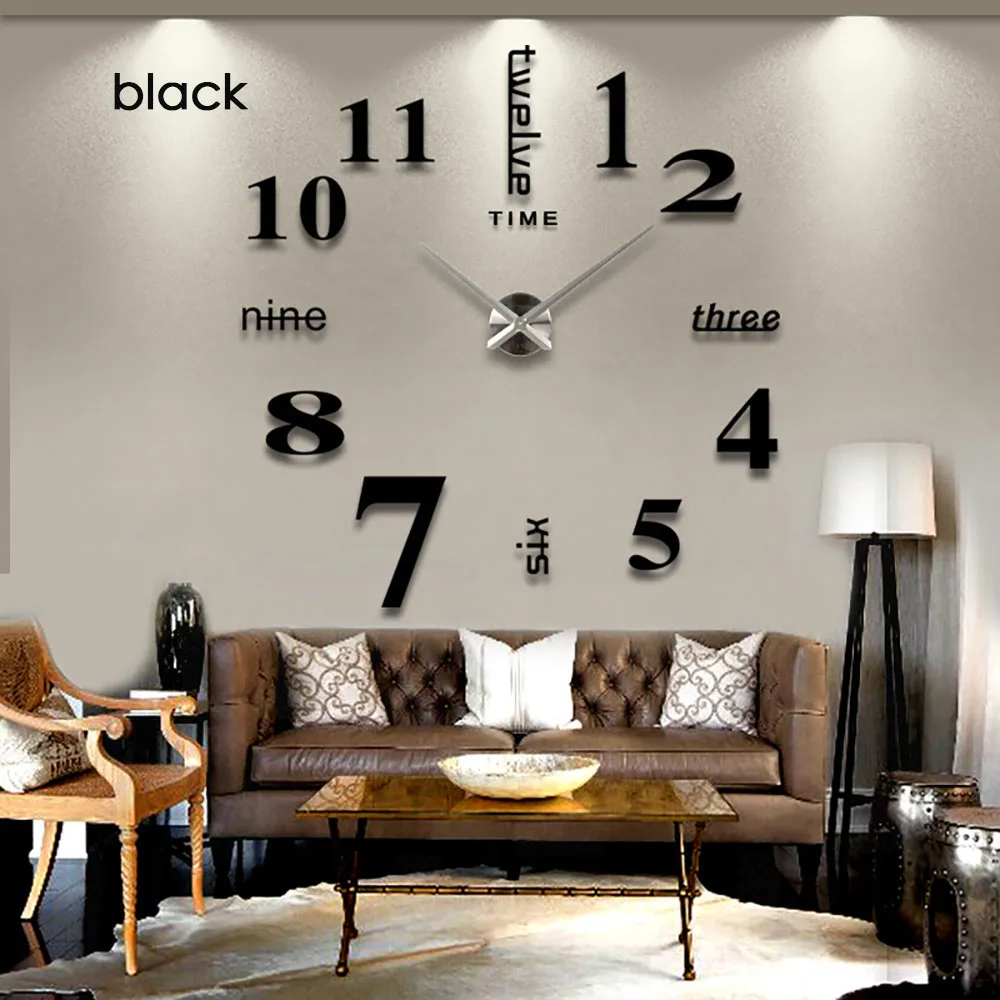This vertical rectangular image depicts a modern living room with a distinctive, wall-mounted clock serving as a prominent feature. The clock spans the entire light gray wall and features silver hands set in the center, surrounded by a mix of black numerals and written-out numbers: 12, 3, 6, and 9 are spelled out, while 1, 2, 4, 5, 7, 8, 10, and 11 are numerals, with the numeral 7 being the largest and the numeral 5 the smallest. The word "black" is visible in the upper left corner, possibly referencing the manufacturer.

The room features a brown leather loveseat adorned with three white pillows, positioned against the clock wall. To the right of the loveseat stands a white lamp, while to its left, there is a wooden chair and a small table with a vase. The floor is covered by a white rug, upon which sits a coffee table with brass legs and a possible brass top, holding a white bowl. Above the clock, three recessed lights illuminate the space, highlighting the cozy yet sophisticated decor.